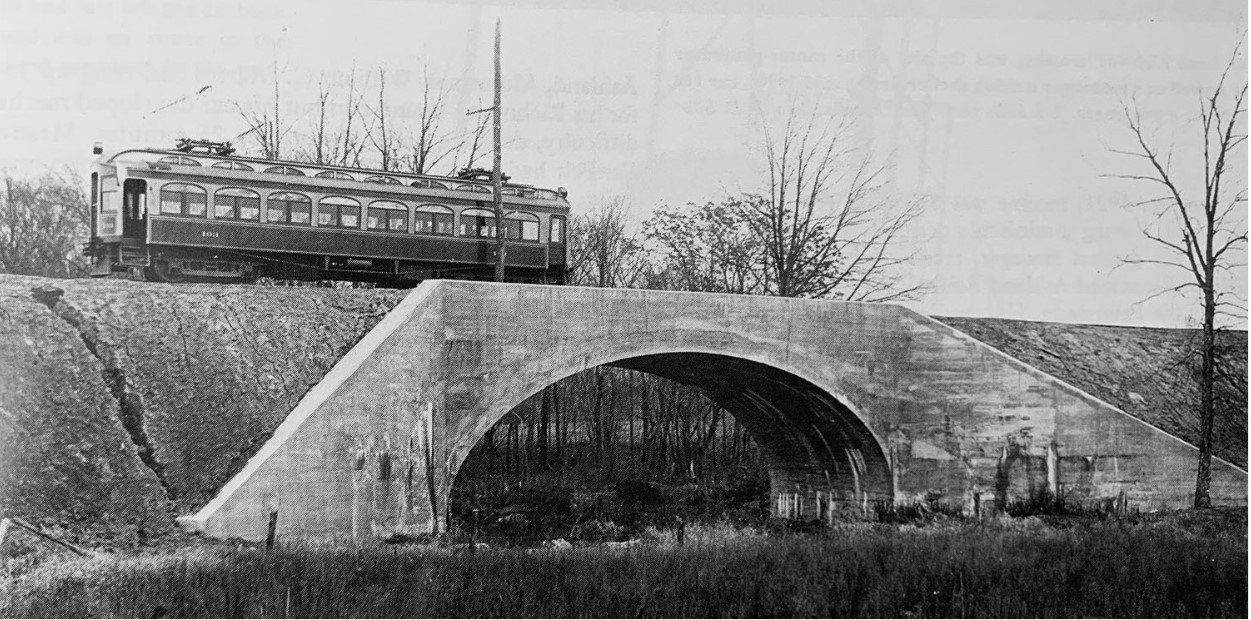In the black and white photograph, a solitary streetcar, resembling a single-cab subway car from the 1950s or 60s, rests on a trestle bridge. The slightly dilapidated streetcar lacks visible overhead cables or tracks, adding to its abandoned appearance. The bridge, constructed from concrete, spans a body of water that is fed by a rounded culvert with a cement outline beneath it. Directly to the right of the culvert opening stands a barren tree, devoid of leaves, its skeletal frame adding to the desolate atmosphere. In the distance, more leafless trees can be seen under an overcast sky, enhancing the grayscale tones of the image. At the bottom of the photograph, dark-shaded grass and a few old fence posts are visible. Moreover, there's a notable crack in the earth embankment on the left. The streetcar’s side door is slightly open, and its windows feature arched tops, hinting at a design that was likely intended to let in ample light.